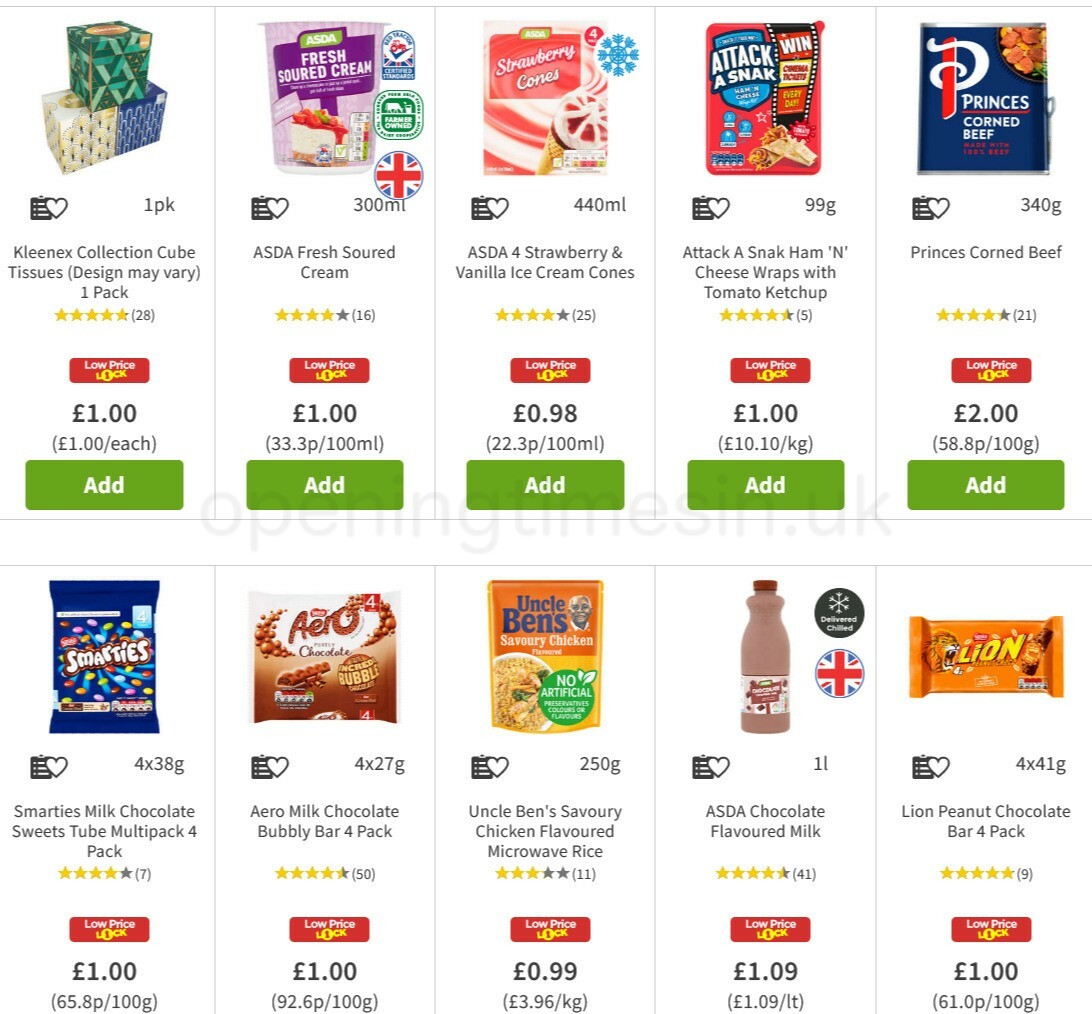Here is the cleaned-up and detailed descriptive caption based on the provided information:

---

The image depicts a screenshot from either an app or a website showcasing a variety of food items available for order. The items are arranged neatly in two rows with five products in each row. Each product is presented with a corresponding image, followed by a heart icon, details about the size, amount, or weight of the product, the product name, a star rating, a "Low Price Lock" indicator in a red box, the price information (including per milliliter cost where applicable), and finally, an "Add" button in a green box for easy addition to the cart.

**Top Row, from left to right:**
1. Kleenex Collection Cube Tissues.
2. ASDA Fresh Source Cream.
3. ASDA Strawberry and Vanilla Ice Cream Cones.
4. Attack and Snack Ham and Cheese Wrapped with Tomato Sauce.
5. Prince's Corned Beef.

**Bottom Row, from left to right:**
1. Marty's Milk Chocolate Sweet Tubes Multi-Pack (4-pack).
2. Aero Milk Chocolate Bubbly Bar (4-pack).
3. Uncle Ben's Savory Chicken Flavored Microwave Rice.
4. ASDA Chocolate Flavored Milk.
5. Lion Peanut Chocolate Bar (4-pack).

Each item is clearly displayed with comprehensive details to assist users in making informed purchasing decisions.